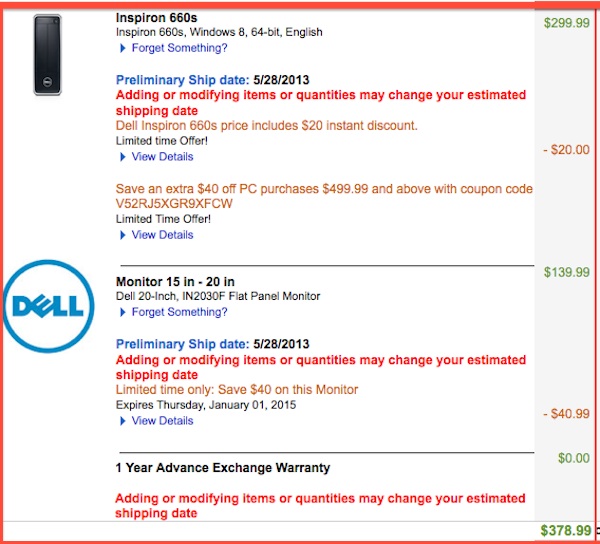The image depicts a webpage for Dell products, specifically showcasing the shopping cart of a customer. At the top, the Dell Inspiron 660s—a Windows 8 64-bit English computer—is highlighted. A notification prompts the user with "Did you forget something?" allowing for adjustments to their cart order. The page displays pricing details on the right side, confirming that this is indeed a shopping cart review before checkout.

The preliminary ship date for the Inspiron 660s is estimated to be May 28, 2013, with a note that altering items or quantities may affect this date. The price for the Inspiron includes a $20 instant discount, which is currently a limited-time offer. Initially priced at $299.99, the discount reduces the cost by $20.

Additionally, the cart includes a Dell flat-panel monitor, specifically a 20-inch model with the product number INF Tool 30F, priced at $139.99. This item also mentions a preliminary ship date of May 28, 2013, and includes a limited-time discount of $40.99. 

The order comes with a one-year advanced exchange warranty at no extra charge. Modifying the items might change the shipping date, as reiterated at the bottom of the page. The grand total for the cart is displayed as $378.99.